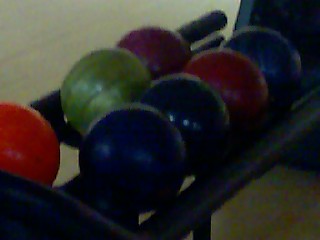The image depicts a low-quality, enlarged thumbnail close-up of a bowling ball rack under dim lighting, making the details fuzzy and blurry. The bowling balls, which appear almost identical in size, are placed on a black rack with tube-shaped sides and supported by black legs. The rack holds seven bowling balls: starting from the left, there's a partially visible reddish-orange ball, followed by a lime green, a magenta or bright purple, a dark blue, a black or dark gray, a maroon or dark red, and another dark blue or navy blue ball. Slight reflections of light are visible on the tops of the balls. The floor beneath the rack, though mostly indistinguishable due to the blur, appears to be cream-colored.